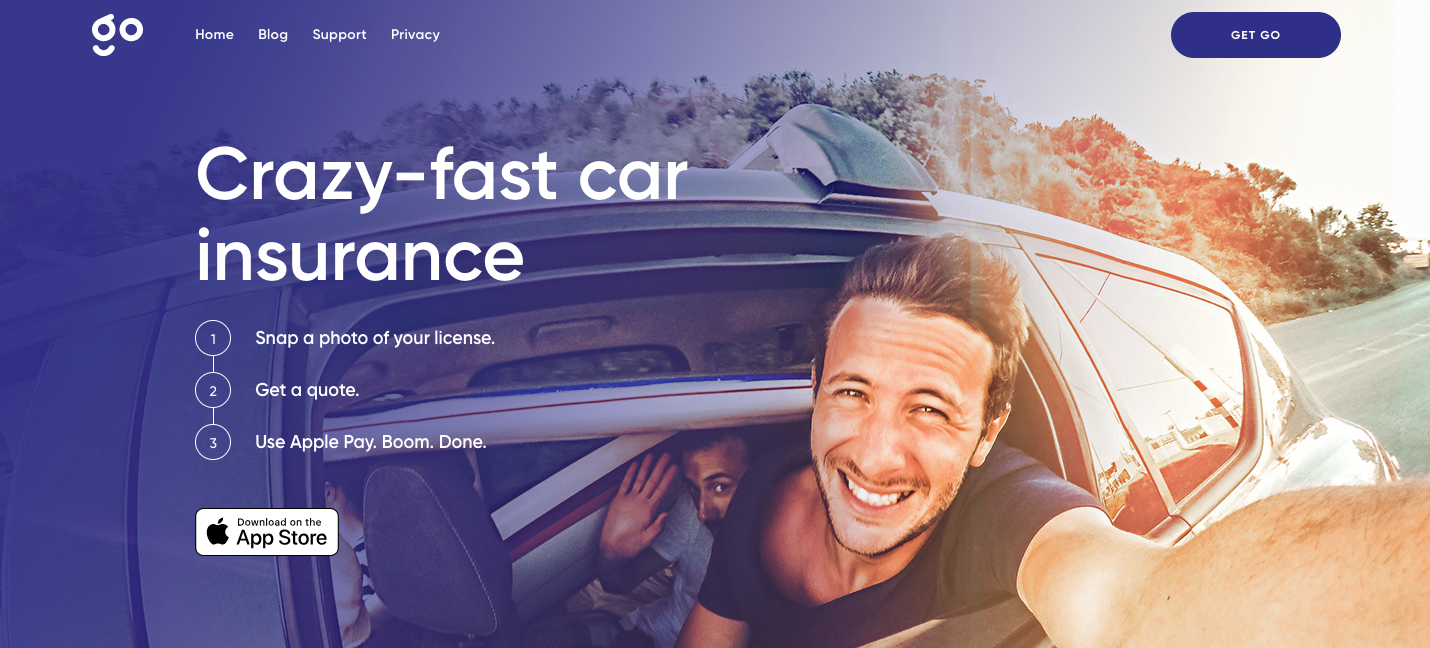A vibrant web advertisement captures the essence of a carefree and adventurous road trip, set against a calming blue background. At the top of the ad, the bold website name "Go" is prominently displayed, alongside navigational links: Home, Blog, Support, Privacy. The eye is drawn to a high-energy photograph featuring a euphoric man leaning out of a car's passenger window on the driver's side, his head thrown back in laughter as he snaps a selfie with his phone. Behind him, surfboards are visible, suggesting a fun-filled journey in the sun. Below the image, dynamic text reads "Crazy Fast Car Insurance," perfectly matching the car's speedy momentum. A call to action invites users to "snap a photo of your license and get a quote," and emphasizes the ease of using Apple Pay with "boom, done." The advertisement concludes with a prompt to download the app from the Apple Store, encapsulating the straightforward, exciting experience of using "Go."